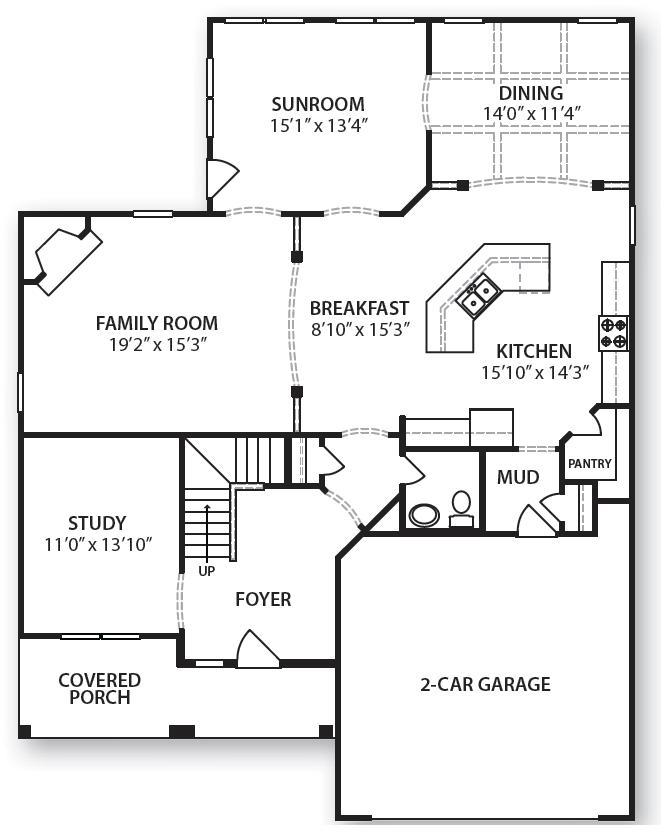This set of blueprints illustrates a detailed top-down layout of the ground floor of a house, meticulously measured and labeled. Starting from the top, which represents the front of the house, there is a spacious sunroom measuring 15 feet by 13.5 feet. Adjacent to the sunroom on the right is the dining room, with dimensions of 14 feet by 11 feet 4 inches.

Proceeding downwards in the blueprint, the house opens into a generous family room, which spans approximately 19 feet by 15 feet, accommodating a variety of family activities. To the right of this area lies the breakfast nook, sized at 8 feet by 15 feet, and next to it, the kitchen, which is 15 feet by 14.5 feet, designed to support culinary endeavors and casual dining.

Toward the lower portion of the layout, on the far left, is a study covering 11 feet by 13 feet, ideal for a home office or quiet reading space. Adjacent to the study is the foyer, though its dimensions are unspecified, featuring an entryway that likely includes steps leading to the front door.

Additionally, the blueprint details practical spaces, including a mudroom and a pantry, facilitating household organization and storage. On the left side, there is a sizable two-car garage, though its exact dimensions are not provided. Completing the floor plan is a covered porch at the front entrance, also without specified measurements.

Recapitulating, this comprehensive house plan outlines the sunroom, dining room, family room, breakfast nook, kitchen, study, foyer, two-car garage, mudroom, pantry, and covered porch, all within the ground floor layout, idealized for functional and comfortable living.